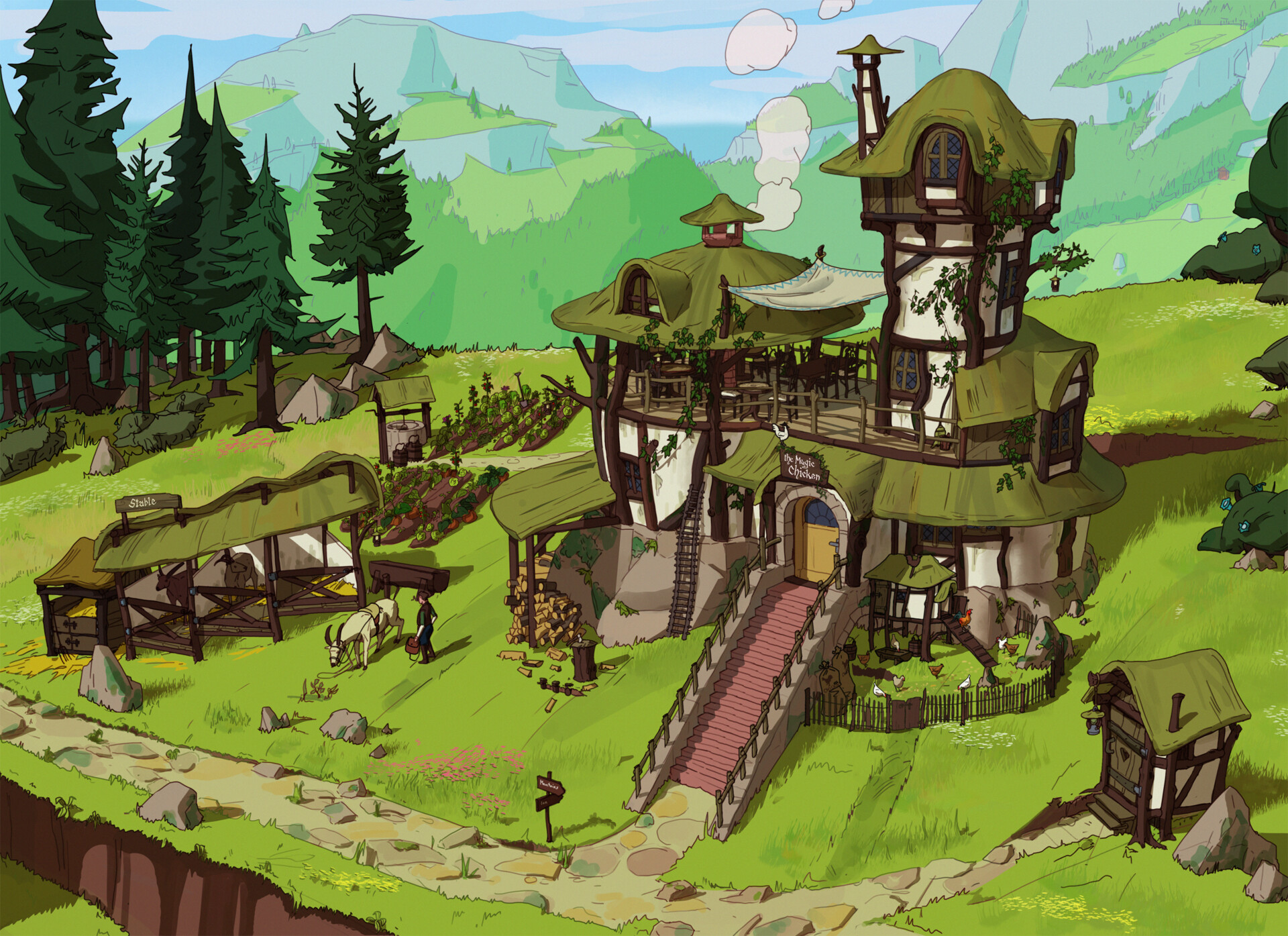This image depicts an animation-style, cartoon-like scene featuring a quaint village setting surrounded by natural beauty. In the foreground, a gently sloping hill is covered with lush green grass, hosting a single, two-story house that evokes the feel of a treehouse, with a light white façade and brown wooden trim. The house boasts a green roof, red steps bordered in gray, and an arch-shaped door. Adjacent to the house is a stable with a green roof, and grazing nearby is a goat or ram. 

To the left of the house, a cluster of pine trees is interspersed with rocks. A stone pathway meanders through the scene, leading to an outhouse situated in the front yard. The background presents a picturesque landscape with rolling green mountains and a bright blue sky, adorned with wispy clouds. Smoke curls from the house's chimney, adding a cozy touch to the idyllic setting. A signpost with wooden arrows directs visitors either straight ahead or towards the house, enhancing this charming, picturesque scene.